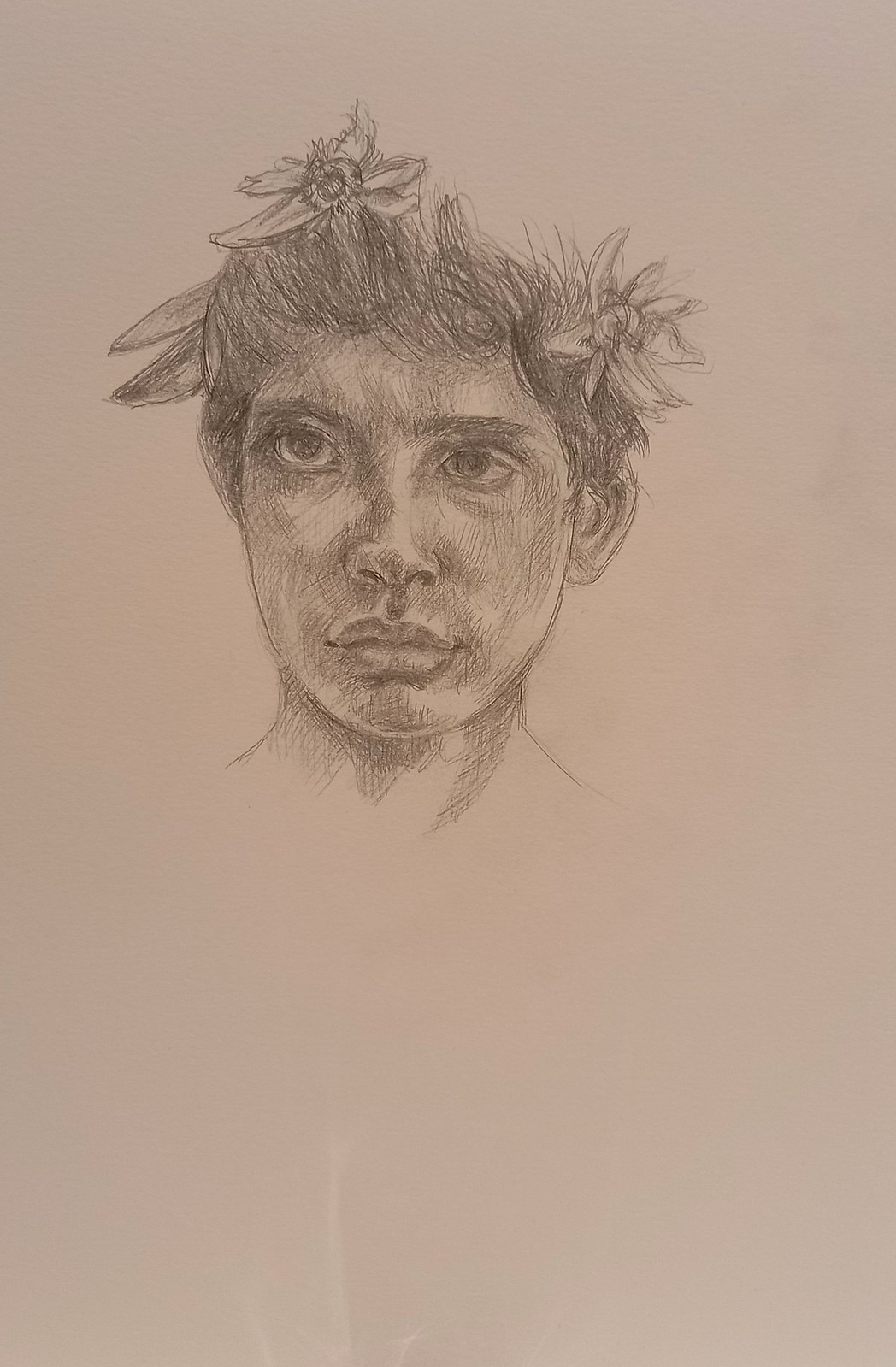This is a detailed pencil drawing on grayish-pink colored paper, depicting a youthful individual whose gender is ambiguous. The portrait extends from the top of the head to just below the chin, showing only a partial portion of the neck. A subtle shadow is skillfully placed beneath the chin, adding depth and realism to the artwork.

The subject's hair is dark and short, almost boyish in style, but adorned with several flowers, which might suggest femininity. The facial features include thick eyebrows, large expressive eyes, an average-sized nose, and full lips. The shape of the face is oval. Despite the detailed rendering, the drawing does not provide enough information to determine the person's race. The combination of a floral element in the hair and the androgynous facial features creates an intriguing and thought-provoking portrait.